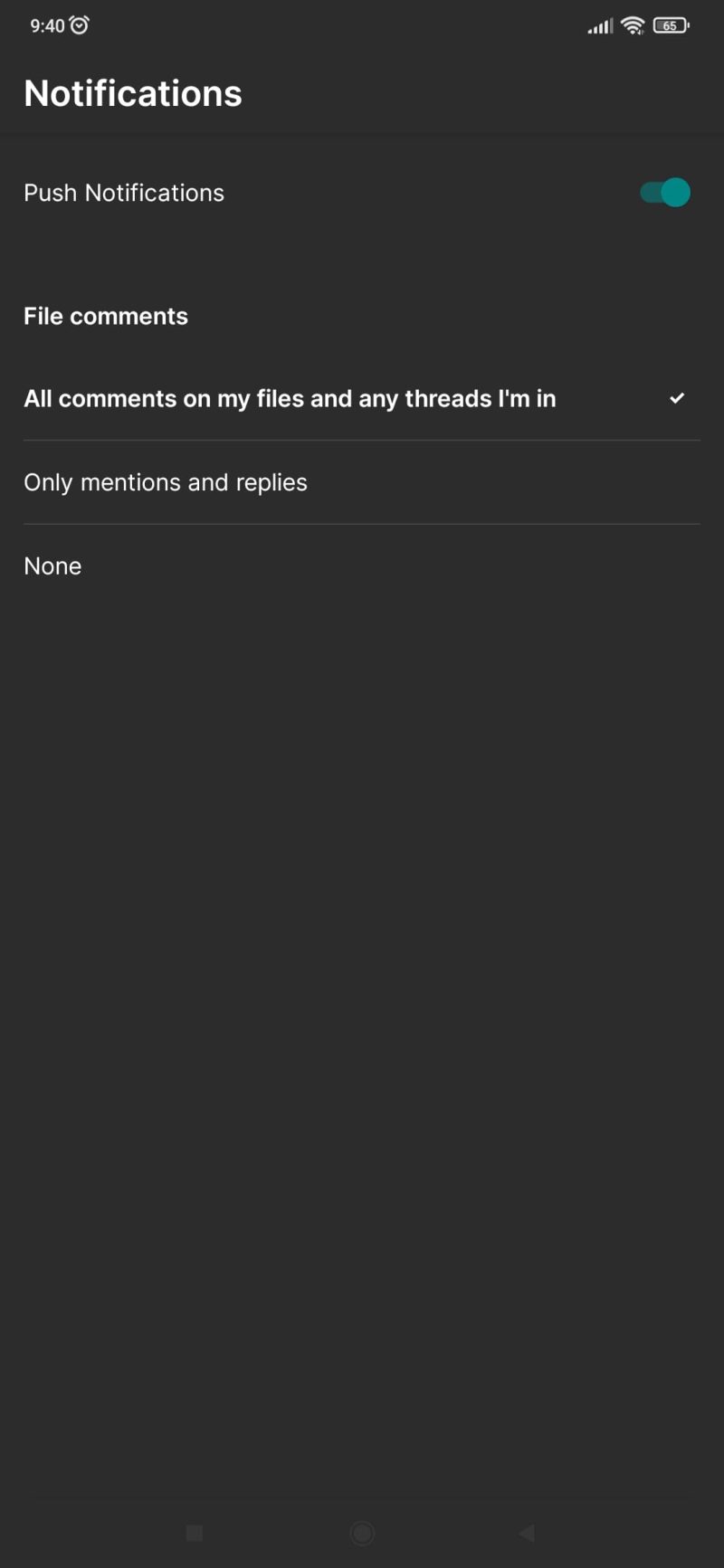This is a detailed screenshot from a smartphone with a predominantly black background and a vertically elongated rectangular shape. The top left corner displays the time "9:40" in white. Adjacent to the time, on the right side, an alarm icon is depicted. Continuing to the right, the battery icon appears in shades of gray and black, indicating a 65% charge with a white outline. To the left of the battery icon, the Wi-Fi symbol is shown at full strength, while the internet signal strength is displayed with three of the four bars in white and the remaining one in gray.

On the left side, prominently in large, bold white letters, the word “Notifications” is displayed. Below this heading, in slightly smaller white text, it says “Push notifications,” accompanied by a teal blue toggle switch on the right side, indicating that the push notifications are enabled.

Further down, a small gap separates the next section. On the left, in bold white text, it says "File comments." Directly below it, smaller white text reads "All comments on my files and any threads I'm in," with a white checkmark on the right side indicating this option is selected. Underneath this, a thin gray line precedes the text “Only mentions and replies,” followed by another gray dividing line and the text “None.”

The lower third of the image is mostly blank, except for a vague, light gray circle faintly visible in the center at the bottom. To the left of the circle is a light gray square, and to the right is a light gray triangle pointing to the left.